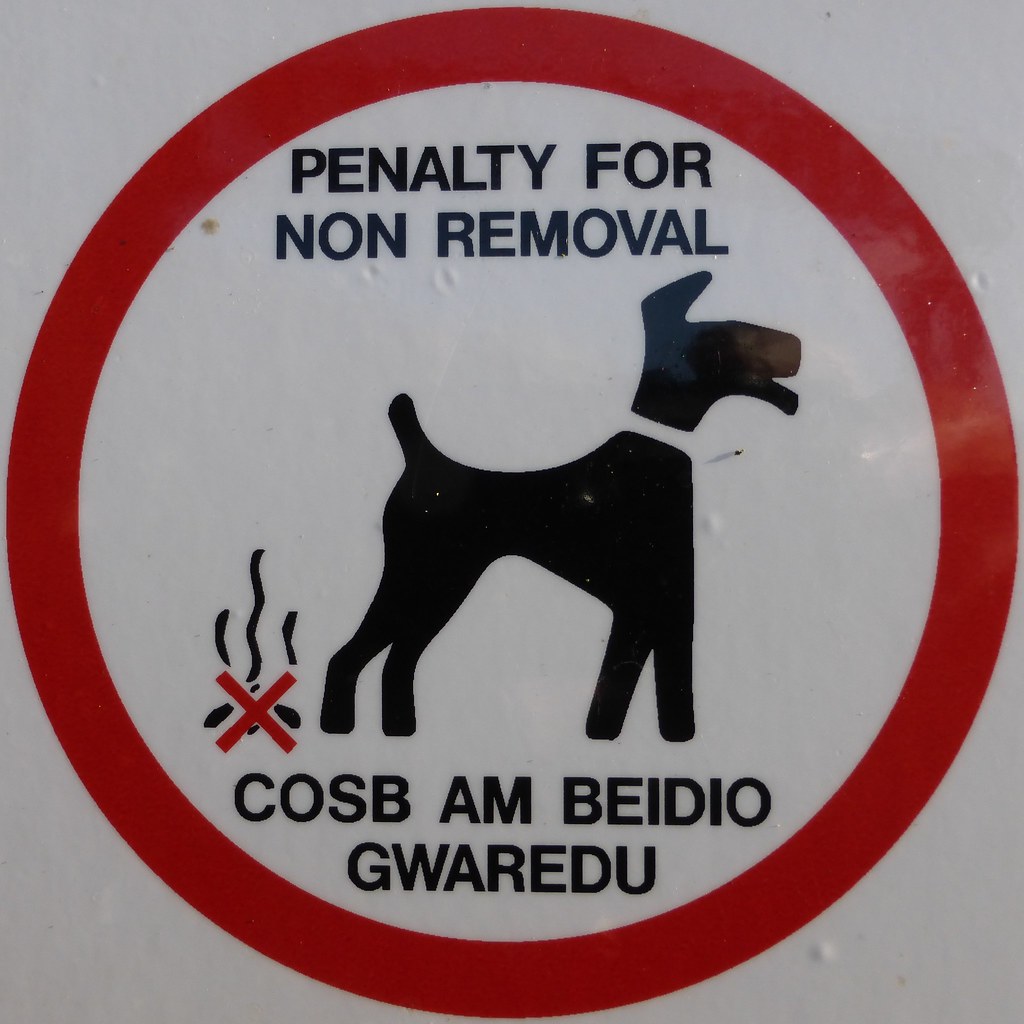The image depicts a street sign with a clear and stern warning about the consequences of not picking up after your dog. The sign features a white background with a large circular red border. At the top, in black letters, it states "Penalty for Non-Removal of Dog Waste." Below the text, centered within the sign, is a silhouette of a dog with its waste depicted on the lower left side, accentuated with stink lines. Covering the image of the waste is a bold red X, indicating prohibition. The same warning text is repeated at the bottom of the sign in Spanish, ensuring the message is clear to a broader audience. The sign’s intent is unmistakable, urging pet owners to responsibly clean up after their dogs to avoid penalties.